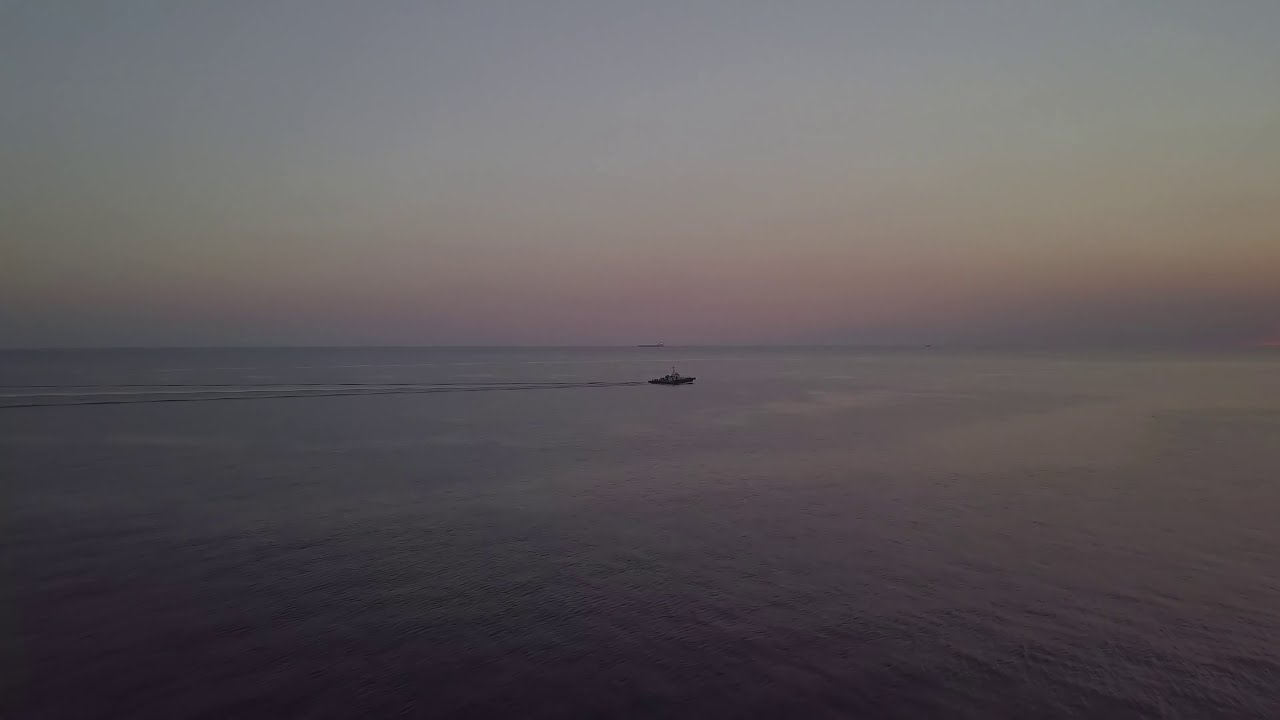In a serene ocean scene, a black and white boat sits in the center of the image, navigating through a vast expanse of calm water. The water's surface, a soothing blend of light and dark blue hues, is dotted with subtle ripples from the boat's wake, which trails behind in delicate waves. In the far distance, where the ocean meets the horizon, a massive oil tanker stretches across, its silhouette barely visible. The sky above transitions from a light blue at the top to a soft orange-red closer to the horizon, casting a gentle glow over the tranquil seascape. With no land in sight, the endless water and textured ripples create a sense of boundless serenity.